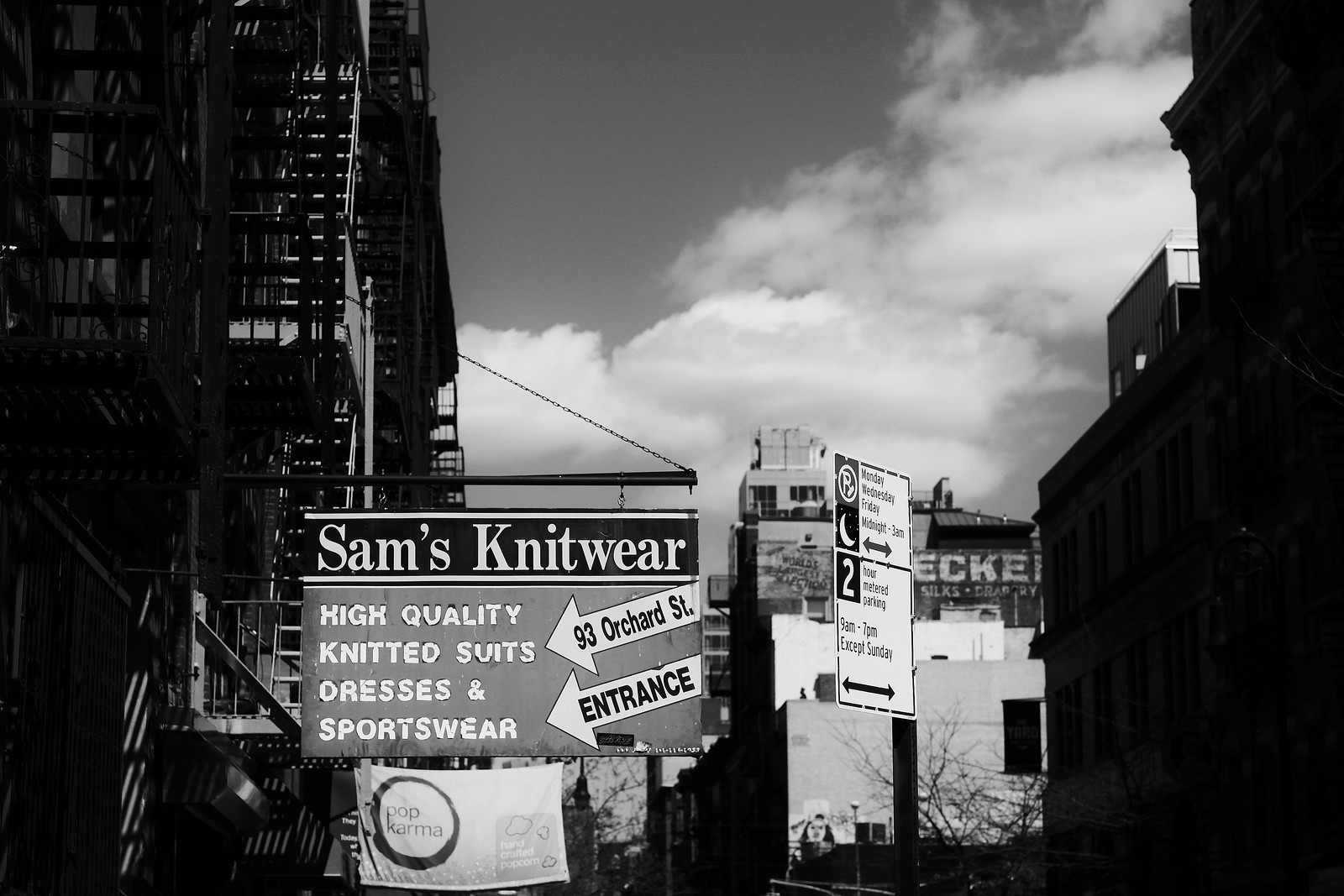The black-and-white photograph captures a busy urban scene, likely taken near an apartment building or similar tall structure. Prominently featured is a sign hanging from the building reading, "Sam's Knitwear: High Quality Knitted Suits, Dresses, and Sportswear," with arrows indicating "93 Orchard Street Entrance." Adjacent to it, there's another sign for "Pop Karma" enclosed in a circle. Additionally, a street sign provides parking information, specifying the hours from 9 a.m. to 7 p.m. On the left side of the image, a fire escape ascends the side of a building, suggesting the photo was taken from the back or side of this edifice. In the background, multiple buildings are visible, one of which has "Decker" written at the top, and there appears to be a billboard or mural depicting a face. The industrial feel, combined with the various signs and buildings, gives the scene a distinctly urban atmosphere.